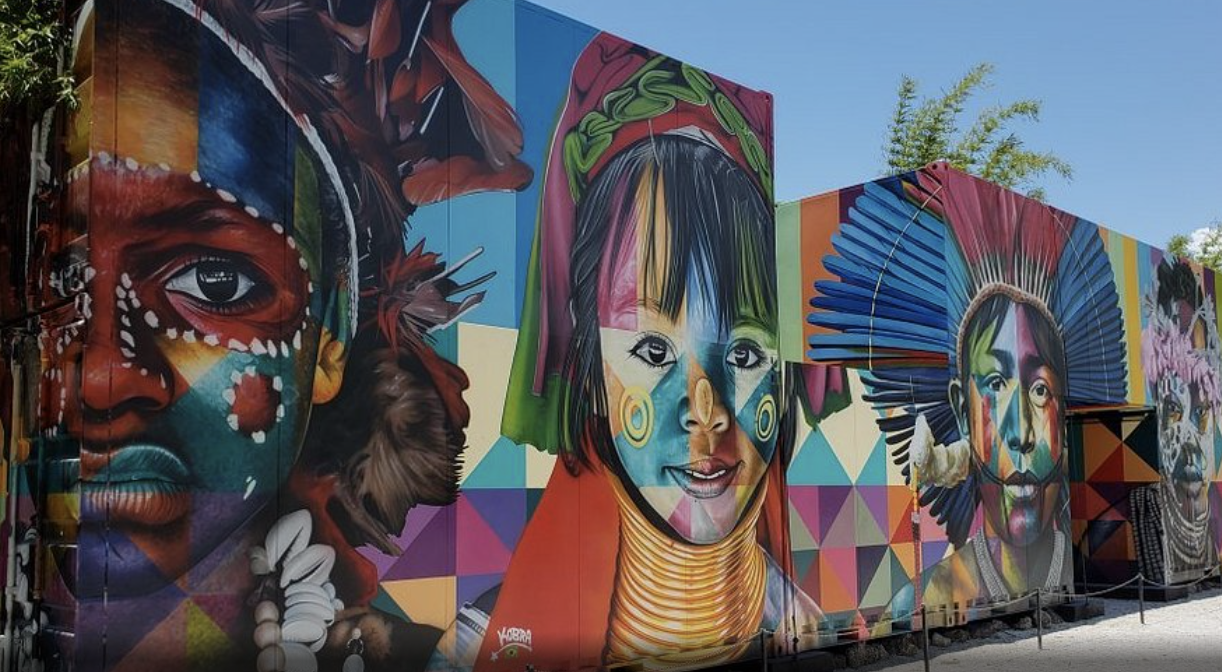The image depicts a vibrant mural on the side of a building, featuring four distinct and colorful portraits of children. Each child’s face is intricately painted in culturally inspired designs. The first child has face paint resembling Native American patterns with a mix of turquoise, purple, red, orange, blue, and green colors. Nearby, the second child is adorned in Aboriginal fashion with a gold neck piece and face painted in sections of blue, orange, bright yellow, pink, light purple, and blue. The third child is decorated in Aztec style with a headdress featuring blue and red feathers, surrounded by backgrounds of colorful triangular shapes. The fourth child exhibits Aboriginal face paint with notable pink hues. The background of the entire mural includes a sky-blue backdrop with a visible tree branch, and the mural is set behind a roped-off sidewalk area to prevent direct contact.